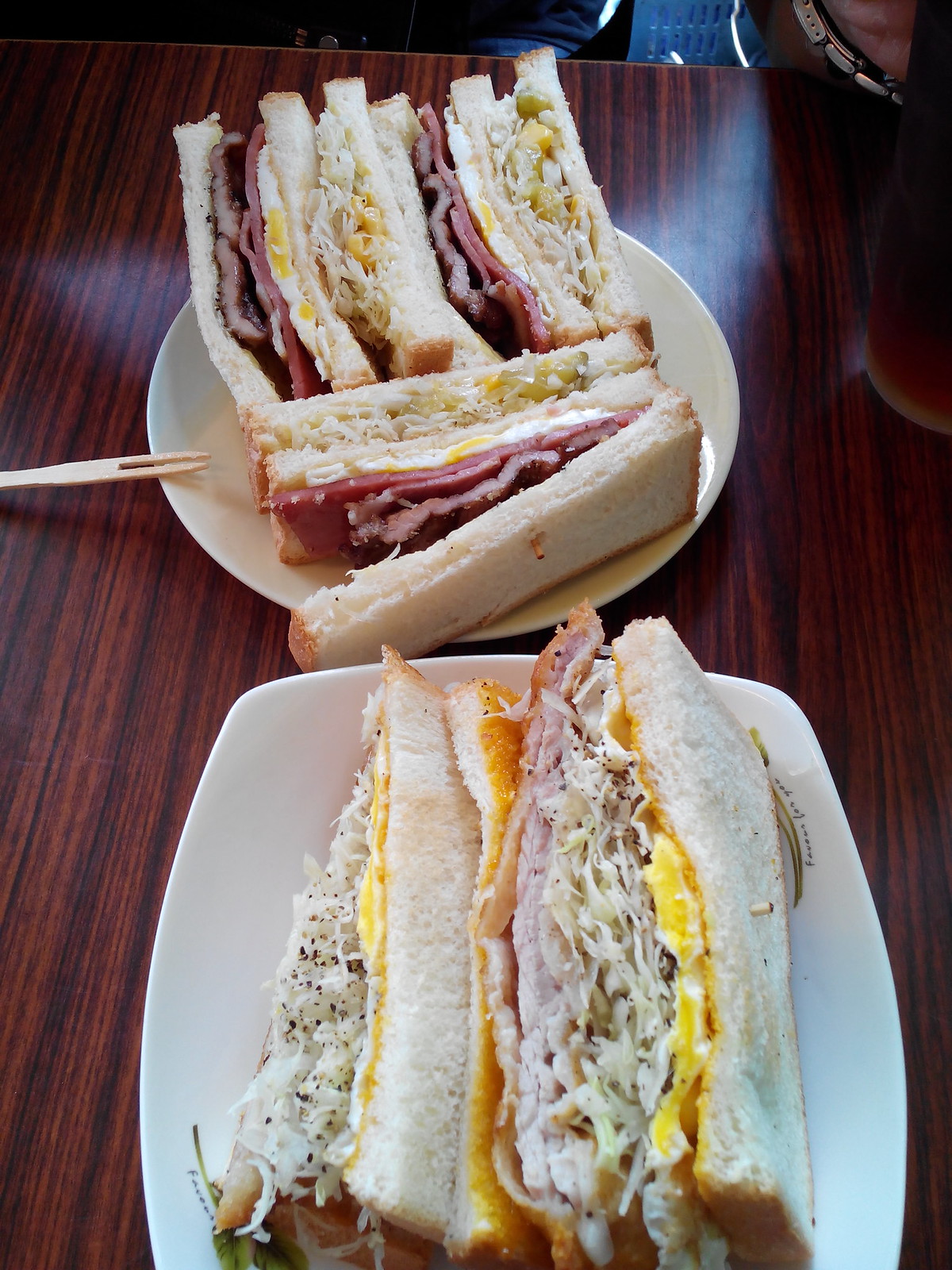This detailed photograph captures a dining scene with two plates of sandwiches arranged on a dark brown wooden table characterized by distinctive black streaks. The top of the frame shows a round white plate with three sandwich halves secured by a wooden two-pronged toothpick. These sandwiches, made with white bread, are filled with a combination of pastrami, eggs, and pickles. Nestled beside this plate is a small, light tan wooden fork.

At the bottom, there’s a squarish round white plate bearing two sandwich halves. This sandwich features white bread enclosing pinkish-colored meat, possibly ham or turkey, along with fried eggs, coleslaw, and a hint of pepper seasoning, all held together with a toothpick.

In the background, a hand wearing a silver wristwatch and some fabric from a dark-colored garment are partially visible. Additionally, a clear glass containing a dark liquid sits towards the right side of the frame. The image exudes a casual dining atmosphere, likely in a restaurant or diner. Overall, the scene combines vivid culinary details with subtle personal elements, capturing a moment of everyday dining.